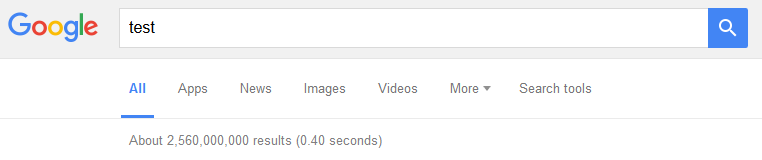The image predominantly features a stark white background with an older version of the Google search interface displayed at the top. The search bar is distinctly rectangular with no rounded edges, adhering to an earlier design style. It is gray, with the actual search input area in white. The iconic "Google" logo is displayed in its classic, colorful font. Within the search bar, the word "test" is typed in lowercase black letters. To the right of the search term is a blue square containing a white magnifying glass icon, indicating the search button.

Below the search bar, the header displays several navigation options. The first link, "All," is highlighted in blue, indicating it is the selected category. The subsequent options, "Apps," "News," "Images," "Videos," "More," (with a drop-down menu), and "Search tools," are all in gray.

Further down, there is an information line in gray text that reads, "About 2,560,000,000 results (0.40 seconds)," conveying the number of search results and the time it took to generate them.